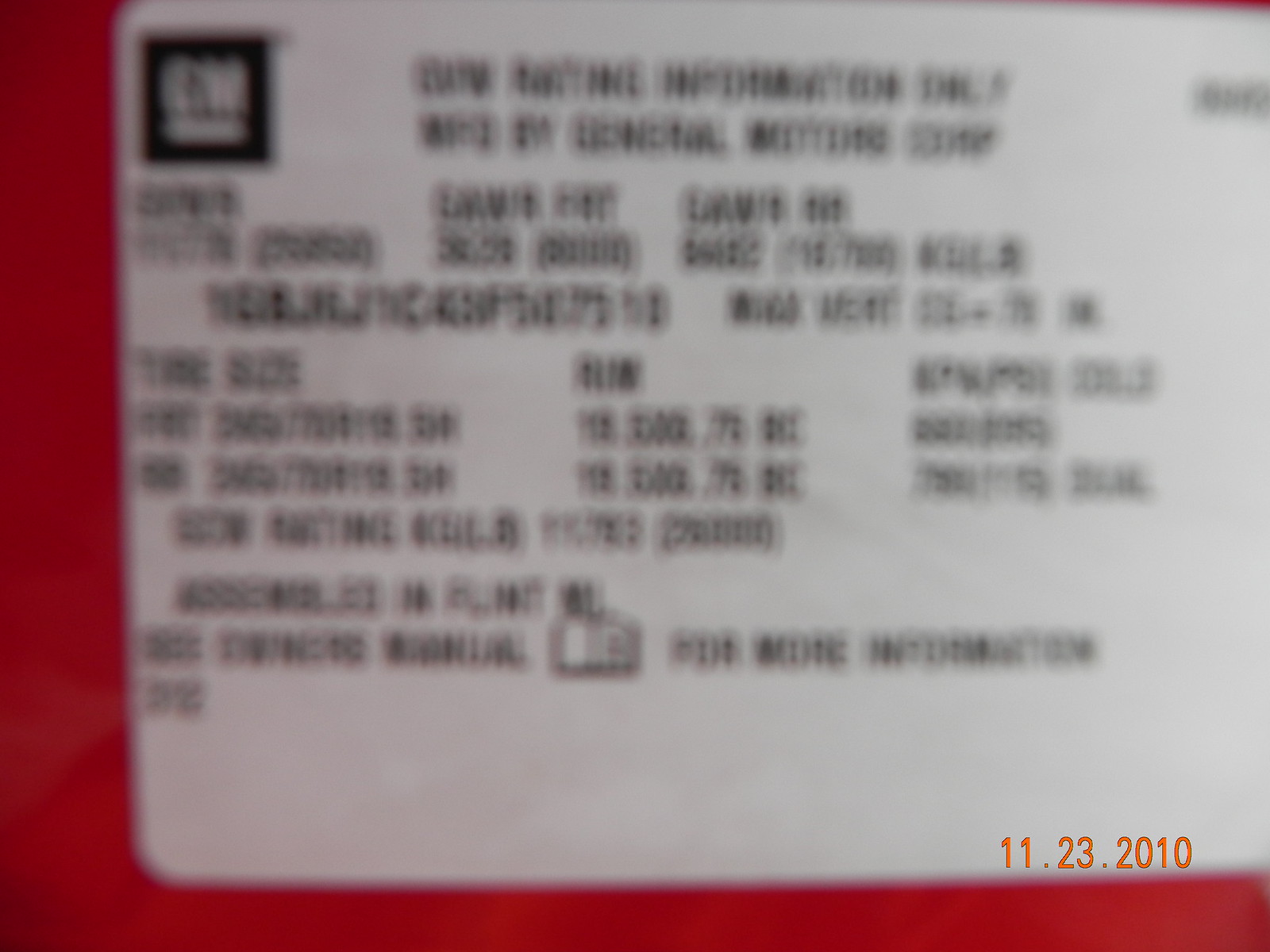This image features a blurred, white label with black text and numbering, situated on a red background. The label bears a date, 11-23-2010, prominently displayed in different accounts as either black or orange text in the lower right corner. In the upper left corner, there is an indistinct black logo that could be interpreted as "CW" or "GM," with an underline or within a black square. The center of the label might contain a sketch that resembles a container. Despite numerous letters and numbers being present, the text is highly unreadable. Columns that potentially include headings like "Time," "Size," and possibly "Altitude" are faintly indicated but not clearly discernible.